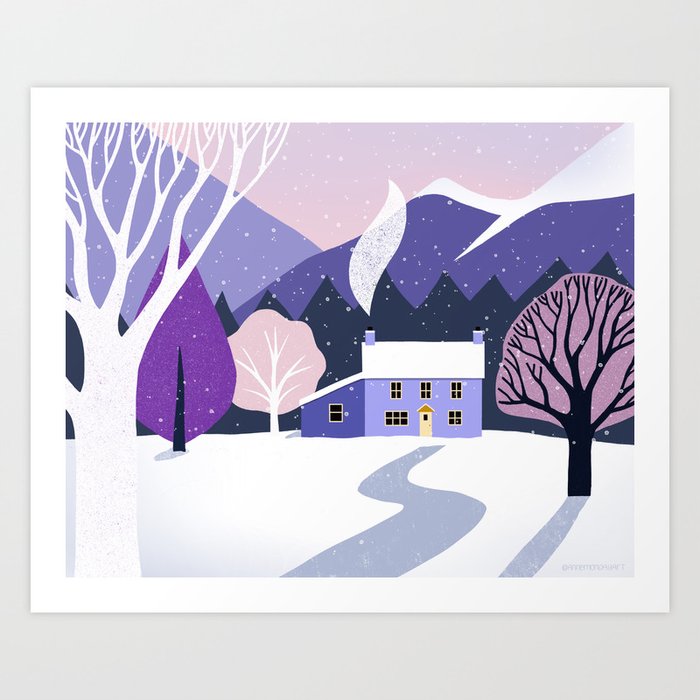This vibrant, cartoon-esque painting illustrates a serene winter scene on what seems to be white cardstock. The central focus is a charming purple house with a distinctive yellow door and two chimneys emitting plumes of white smoke, suggesting a cozy fire inside. The house is detailed with white-framed windows, and a roof blanketed in snow, set against a backdrop of risen, gray, and purple mountains topped with snow. The sky is an unnatural yet tranquil pale pink, speckled with falling snowflakes. 

In the foreground, there is a white, leafless tree prominently positioned on the left, with three additional trees depicted in hues of purple, pink, and black. The snow-covered pathway meanders towards the house, curling through a large white lawn laden with snow. Various colored trees and jagged formations, rendered in dark blue, purple, and black tones, lend depth to the composition. Gray shadows enhance the wintery atmosphere. The overall palette of purples, pinks, and whites against the soft pink sky creates a tranquil, almost dreamlike quality, richly detailing a picturesque winter wonderland.